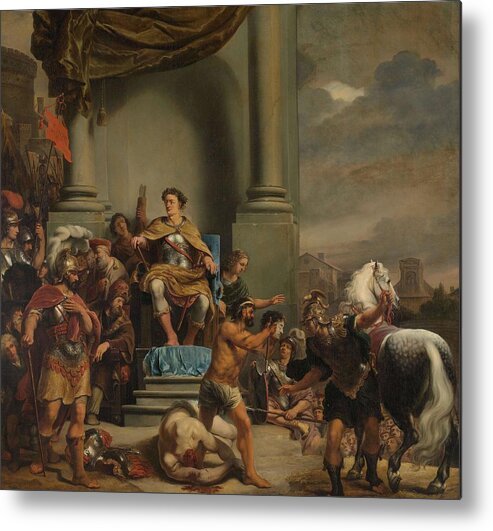The image is an intricately detailed illustration or painting set many centuries ago, portraying a dramatic and somber scene from ancient Rome. The central figure, likely a leader, is seated on an elevated stone throne with three steps, dressed in brass Roman armor and a flowing cape, and gazing sternly to his left. The scene is grim, with a darker tone highlighting its intensity. Surrounding the leader are roughly ten individuals dressed in traditional metallic helmets, long boots, and gladiatorial attire. In front of the throne, a chaotic fight scene unfolds: one Roman soldier stands gripping a horse's rope, the animal displaying a striking black and white coat, while another soldier holds the severed head of his opponent, whose lifeless, pale body lies sprawled on the ground. The background is marked by ominous dark clouds and the partial structure of ancient columns, indicating a setting that is both indoor and outdoor. All present are fixated on the brutal display, adding to the painting's overall tension and historical authenticity.